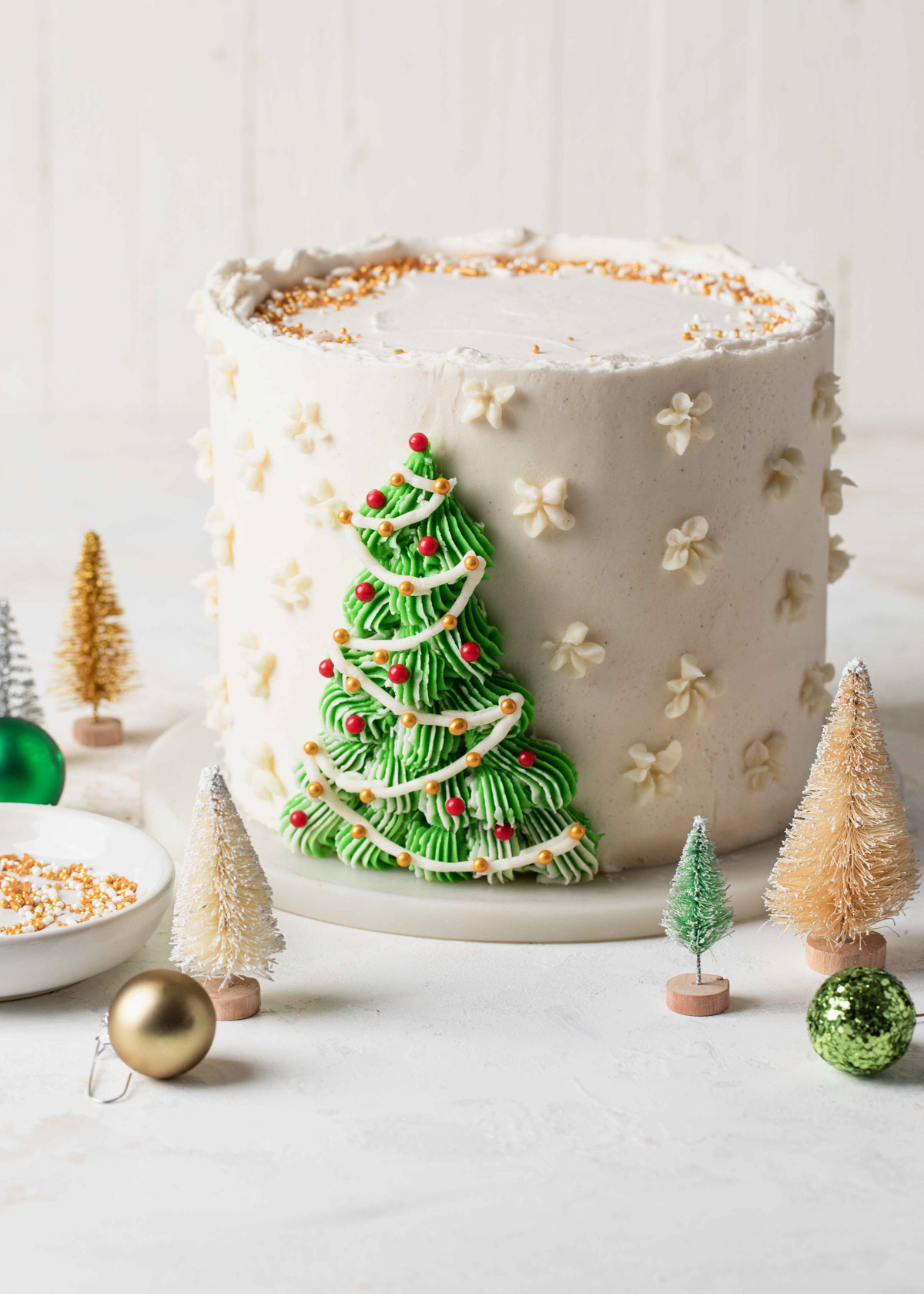The photograph features a strikingly decorated Christmas cake placed on a white surface, which appears to be a tablecloth, set against a white wall background. The cylindrical cake is elegantly simple, primarily white with intricate decorations. At the center of the cake's front, a beautifully frosted Christmas tree stands out, adorned with red and golden beads mimicking ornaments, and possibly shapes resembling flowers or festive decorations. The top edge of the cake is sprinkled with gold and white glitter, adding a touch of sparkle.

Surrounding the cake on the surface are mini decorative pine trees in various colors: silver, gold, off-white with frosting, green with white frosting, and tan. There are also three Christmas ornaments, including a golden one on the lower left, a shiny green bumpy one on the lower right, and another green one partly hidden on the left behind a bowl. The bowl contains the same gold sprinkles used to garnish the cake, tying the whole festive scene together seamlessly.